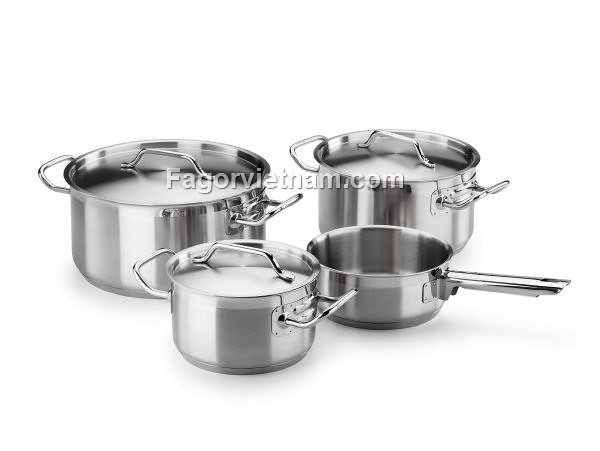In this photograph set against a pure white background, four metal cookware pieces of various sizes are meticulously arranged. The top-left corner features a large, tall, and wide aluminum stock pot with two metal side handles and a metal lid topped with a silvery handle. Adjacent to it, in the top-right corner, is a slightly smaller version of the same stock pot, similarly equipped with side handles and a metal lid. Positioned in the bottom-left is an even smaller pot of the same type, also adorned with side handles and a matching metal lid. Finally, in the bottom-right, there is a small sauce pan with a long handle extending from one side and notably lacking a lid. A semi-transparent watermark, "FAGORVIETNAM.com" in white lettering with a black drop shadow, overlays the image, suggesting its use in an advertisement.